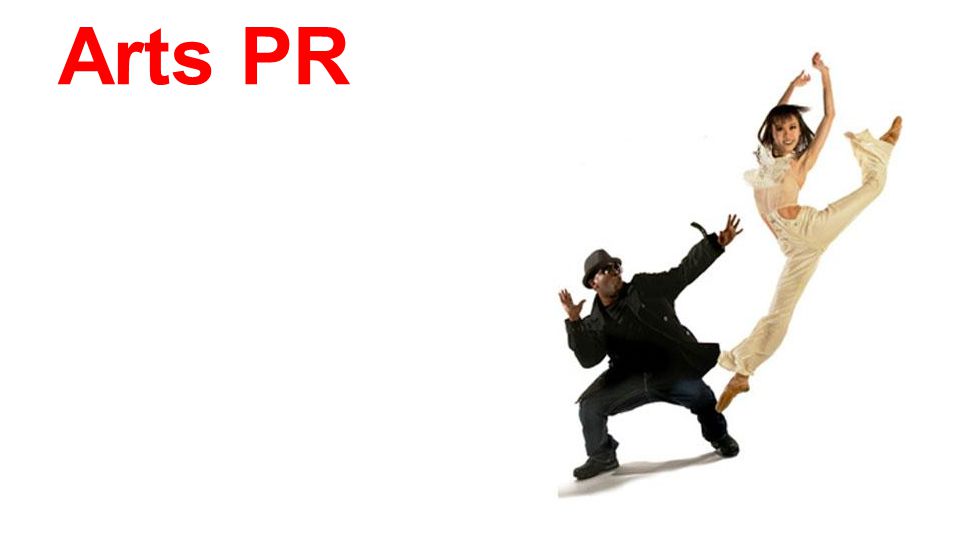In the photograph, set against a stark white background, two dancers captivate the viewer's attention. In the upper left corner, the words "ARTS PR" are prominently displayed in bold red letters. To the left, an African-American man is dressed entirely in black, including a fedora, sunglasses, a long-sleeved denim jacket, jeans, and shoes. His left arm reaches out towards his dance partner, while his right arm is bent at the elbow, pointing upwards.

Adjacent to him is an Asian female dancer, leaping gracefully in a perfect mid-air split. She has thin black hair and wears a white full-body leotard complete with tan ballet shoes. Her arms are elegantly extended above her head, and she gazes directly at the camera. The composition of the image emphasizes a striking contrast between the dancer's black and white attire, adding a visually intriguing element to the captivating scene.